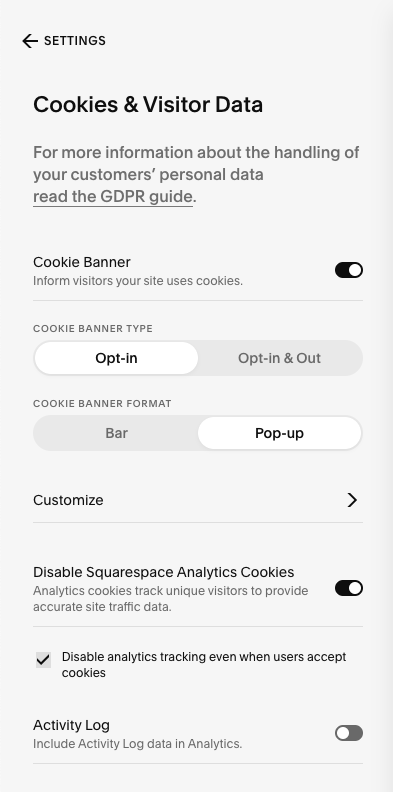The image is a portrait-format screenshot, primarily in black and white. It presents a settings page, likely from a website dashboard or app interface. At the top, a prominent headline in dark black reads, "Cookies and Visitor Data."

Beneath the headline, it provides a brief on GDPR compliance: "For more information about the handling of your customer's personal data, read the GDPR guide." Here, various options related to cookie management can be seen.

A "Cookie banner" option is set to inform visitors that the site uses cookies, marked as 'yes.' The "Cookie banner type" is configured for 'opt-in,' allowing visitors to consent to cookies. The "Cookie banner format" is set to 'pop-up,' which will display a pop-up message to visitors.

An adjacent "customize" button with an arrow suggests further customization options. Below are additional settings, such as "Disable Squarespace Analytics Cookies," which is enabled, and "Disable analytics tracking, even when users accept cookies," which is also activated. The "Activity log" option remains unticked.